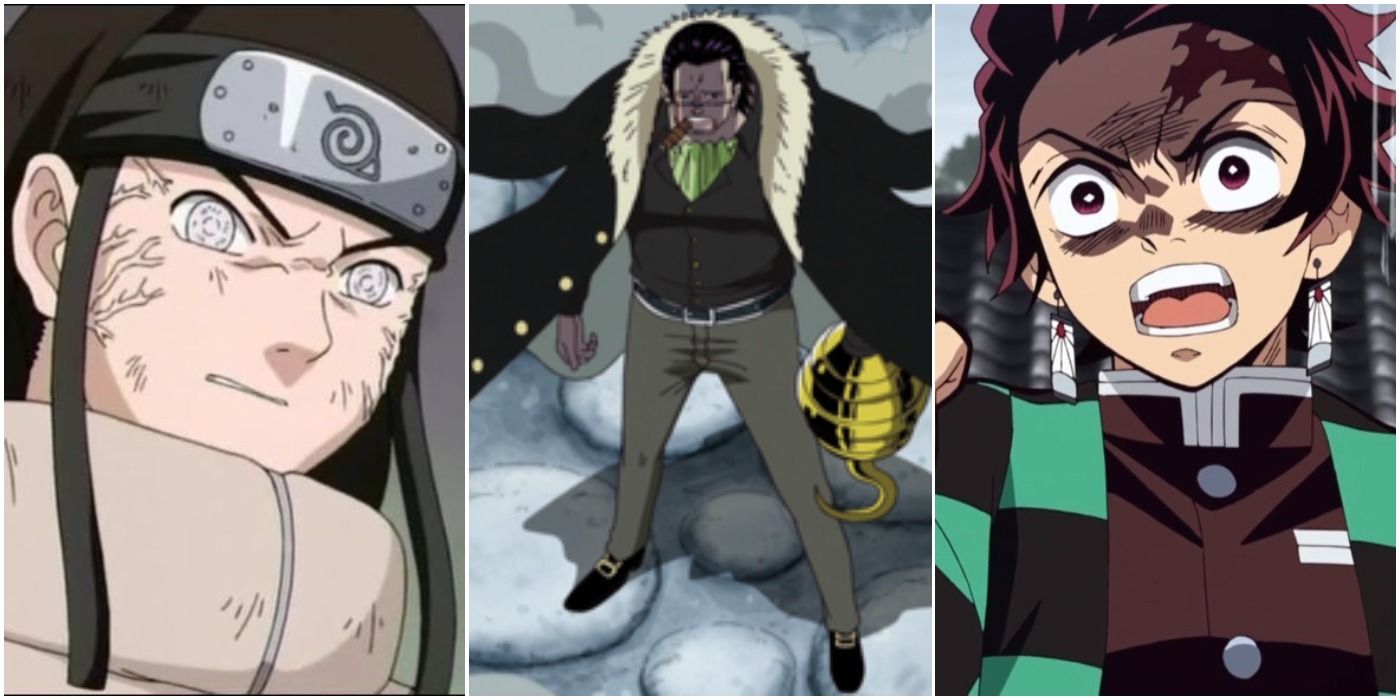The image is a triptych of detailed anime illustrations, each featuring a different male character depicted at varying degrees of intensity and attire. On the left panel, there is a male character with an angry, intense expression, veins bulging on his face. He is dressed in a heavy jacket with a hood, though the visual only extends to his neck. The middle panel showcases a man standing confidently with his legs apart, giving a challenging presence. He wears a large winter coat draped over his shoulders without his arms in the sleeves, exposing a distinctive big hook for a left arm. He also has a cigar in his mouth, glasses, and gray pants. In the right panel, there is another male character who is equally enraged. He has brown hair, brown eyes, and is shouting with his mouth wide open. His eyes are intense, adding to the furious expression on his face. Each character is uniquely detailed, portraying a blend of distinctive visual elements and emotional depth.